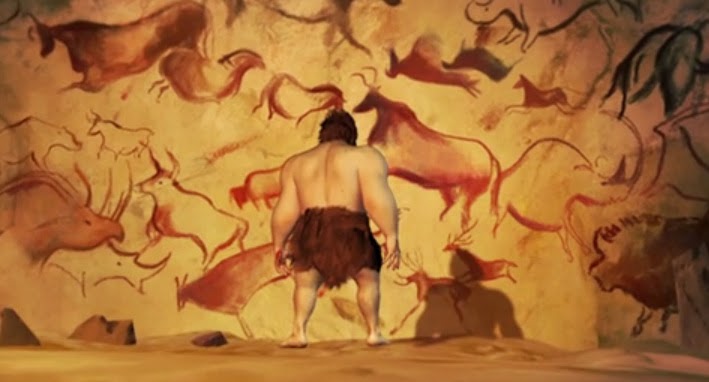In this detailed graphic image, a shirtless, white, computer-generated caveman with long black hair stands barefoot with his back to the camera. He is clad in a brown, animal-skin loincloth that reaches just above his knees. The setting is indoors, depicting the interior of a cave. The cave wall is a vivid mix of brown and orange hues, and it's covered with various animal drawings primarily in brown and some in black. These cave paintings include animals with horns, such as buffalo and rhinoceros-like creatures, in profile. Some of the animals are leaping and running, with detailed features such as a moose-like figure and a boar in the bottom right-hand corner. The caveman casts a shadow on the wall, indicating that the light source comes from the left and is positioned high up. The surface of the cave is sandy with a few rocks scattered, predominantly on the left side of the image. The overall aesthetic of the image makes it resemble a painting, despite it being a computer-generated graphic, capturing a moment where the caveman contemplates these ancient artworks.